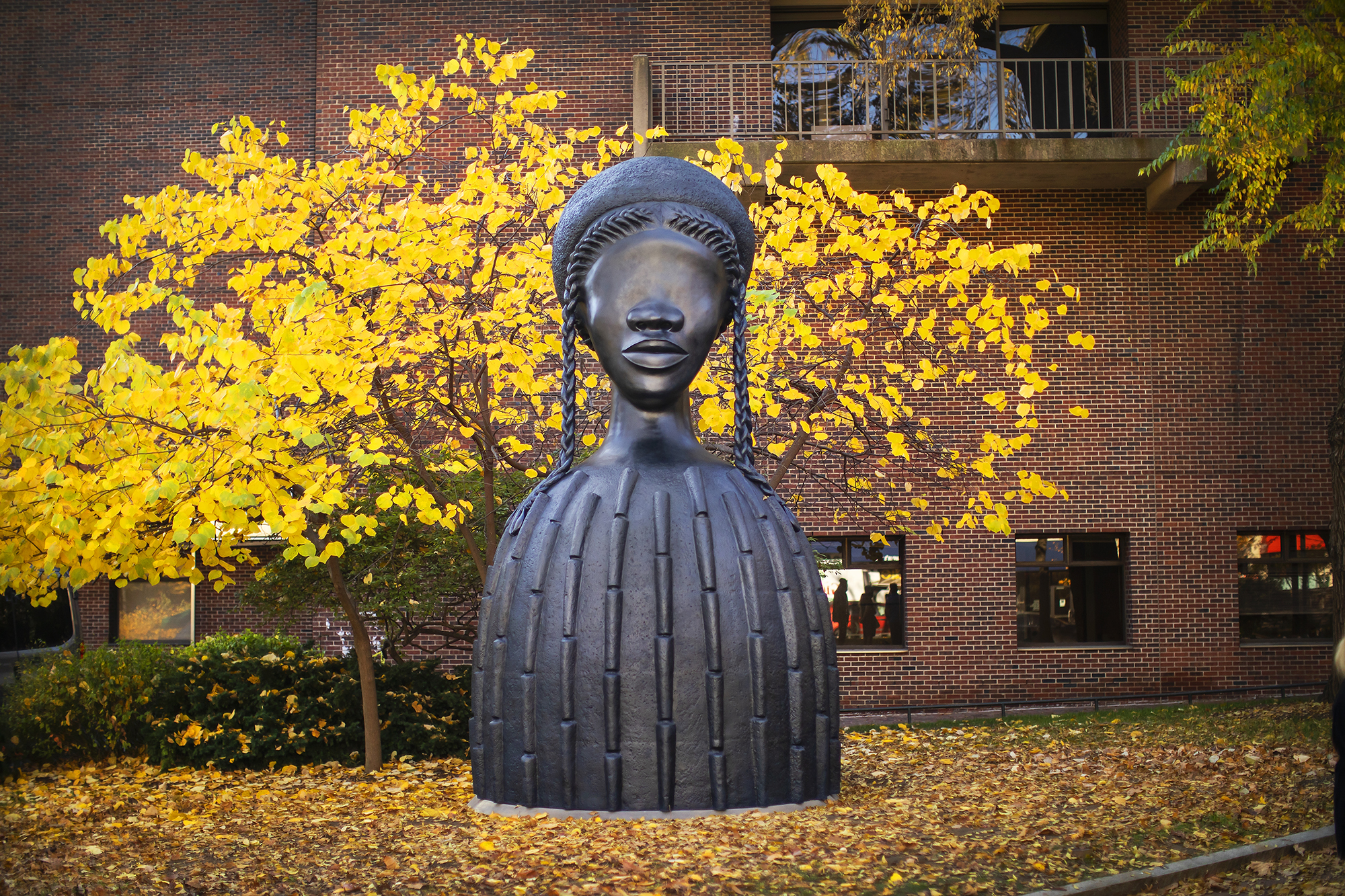In this detailed image, we see a striking outdoor sculpture of an African woman, prominently featured against a fall backdrop. The statue, standing tall and as high as some of the surrounding trees, is entirely black and appears quite new, with a body shaped like a dome or bell that has vertical embossed lines. The figure has no eyes, but distinguishes itself with a wide, prominent nose and full lips. The head is adorned with a round hat and long, thick braids fall gracefully on either side of the face, which is a slightly browner tone compared to the rest of the sculpture's body.

Behind the sculpture, we observe a vibrant autumn scene with a tree displaying yellow leaves. The ground is scattered with yellow and brown leaves, indicative of the season, and a green bush peeks out from below the tree. The setting includes a well-maintained green lawn leading up to a red brick building. This building features a balcony on the second floor and has visible windows on the ground floor, through which the silhouettes of people can be seen. Additional tree branches extend into the frame from the left, adding depth to the composition.